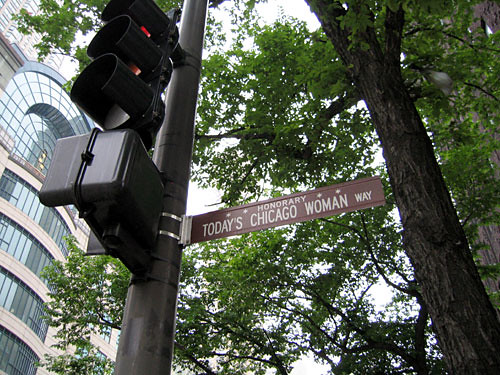This landscape-oriented photograph captures an urban streetscape from a low-angle perspective, focusing upward at a street sign affixed to a light post. The light post, running vertically along the left edge of the image, also supports a brown sign reading "Honorary Today Chicago Woman Way" and a traffic light currently displaying red. On the right side of the frame, a tree of similar thickness to the light post stretches upward, its branches interspersed with green foliage extending across much of the scene and partially obscuring the view. To the left of the light post, a modern glass building features a prominent arched section and curved banks of windows that descend in layers. The background reveals a clear, daylight sky with a subtle whitish hue, enhancing the outdoor ambiance of the urban environment. The scene is well-lit, showcasing the city's architecture and natural elements in harmony.